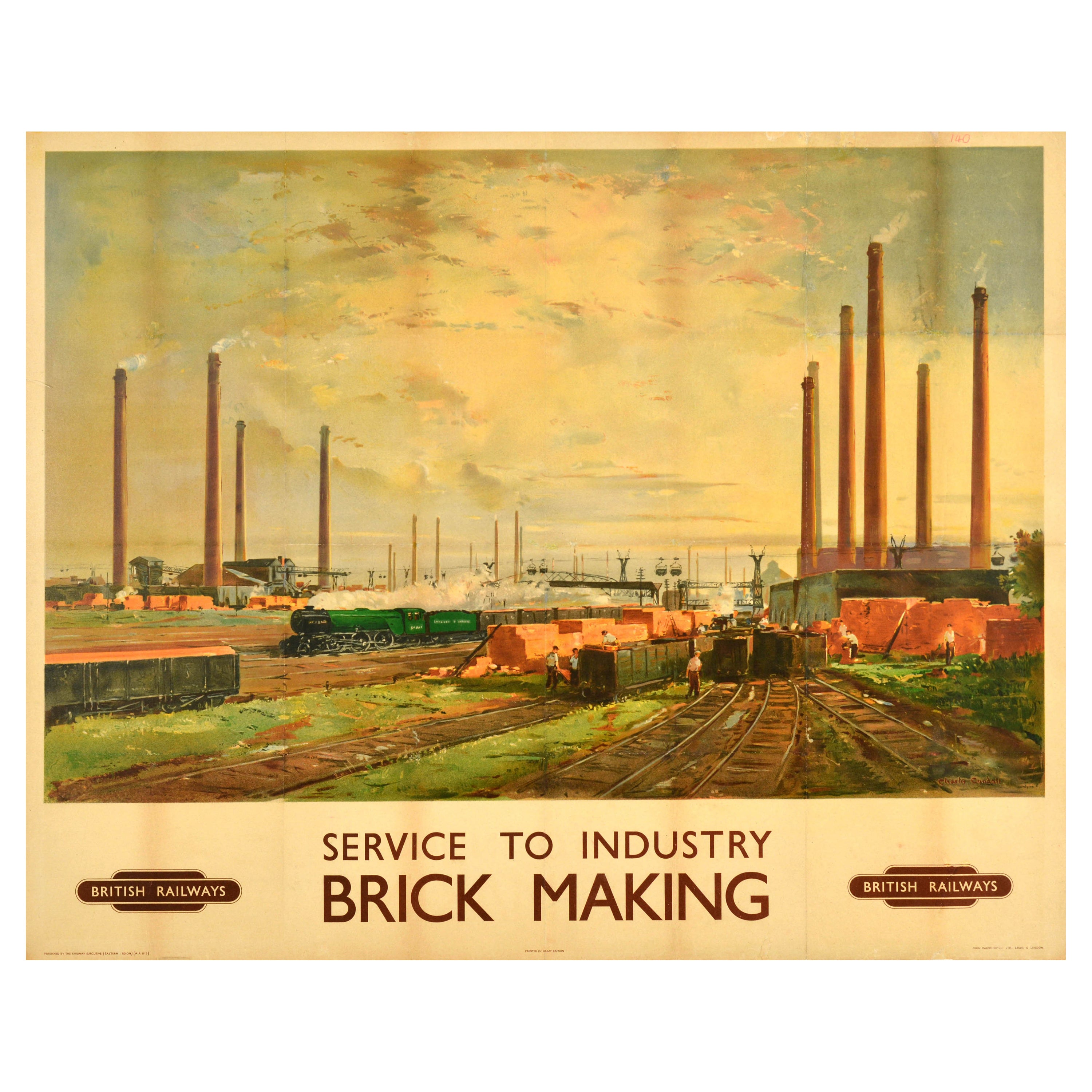This detailed illustration appears on a vintage-style watercolor postcard and depicts a bustling industrial railway yard. The scene is dominated by tall factory chimneys, constructed from orange bricks, spewing smoke into a sky tinged with shades of orange and red. A green and black steam engine hauls rail cars down the tracks, threading through a complex network of six intersecting rail lines. Workers are busily engaged on either side of the tracks, loading and unloading cars adjacent to a green building surrounded by stacks of bricks and large crates of freight.

On the right-hand side of the scene, eight towering, cylindrical stacks rise at least 12 feet into the sky, contributing to the industrious atmosphere. The background reveals more industrial elements and hints of residential areas, with trees and barn-like buildings adding depth to the illustration. 

At the bottom of the postcard, inscribed on a tan background, are the words "British Railways Service to Industry Brick Making," flanked by two British Railways logos. The overall color palette includes fading and muted tones of blue, brown, green, and orange, giving the postcard a nostalgic and weathered appearance.